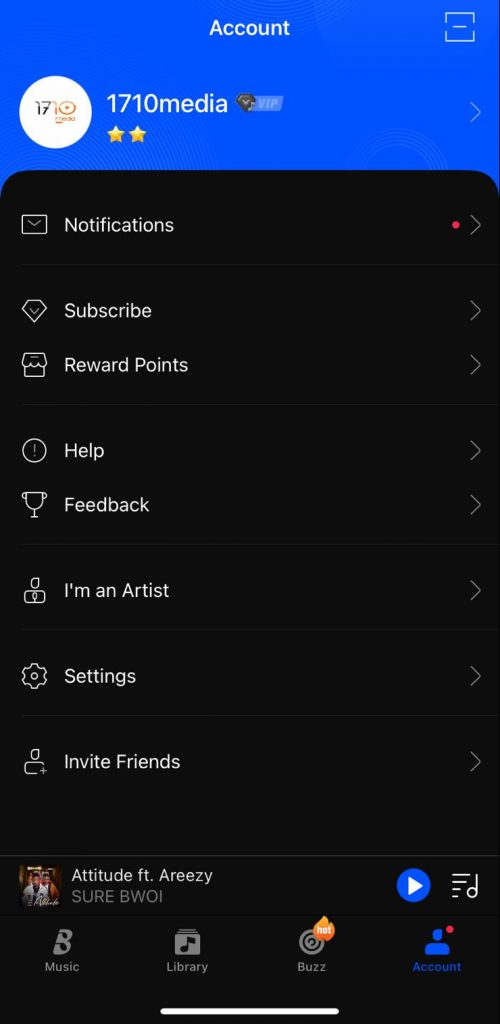The image displays a mobile device showcasing an app interface that isn't immediately recognizable. At the top of the screen, there's a bright blue header with the word "Account" centered in white text. In the upper right corner, there's an icon resembling a nearly complete square with two chunks missing on either side and a horizontal line bisecting it, likely representing a minimize function.

Beneath this header, on the left side, there's a profile icon displayed as a white circle containing the number "1710" with the word "media" below it. Adjacent to this, the text "1710 media" is accompanied by a black diamond shape featuring a checkmark and the label "VIP," with two gold stars directly beneath this label.

The remaining portion of the screen has a black background with various menu options listed in white text: "Notifications," "Subscribe," "Reward Points," "Help," "Feedback," "I'm an Artist," "Settings," and "Invite Friends." There is also a section featuring "Attitude" by artist "Areezy or BWOI," highlighted with a blue play button. Below this, additional categories are labeled "Music Library," "Buzz," and "Account."